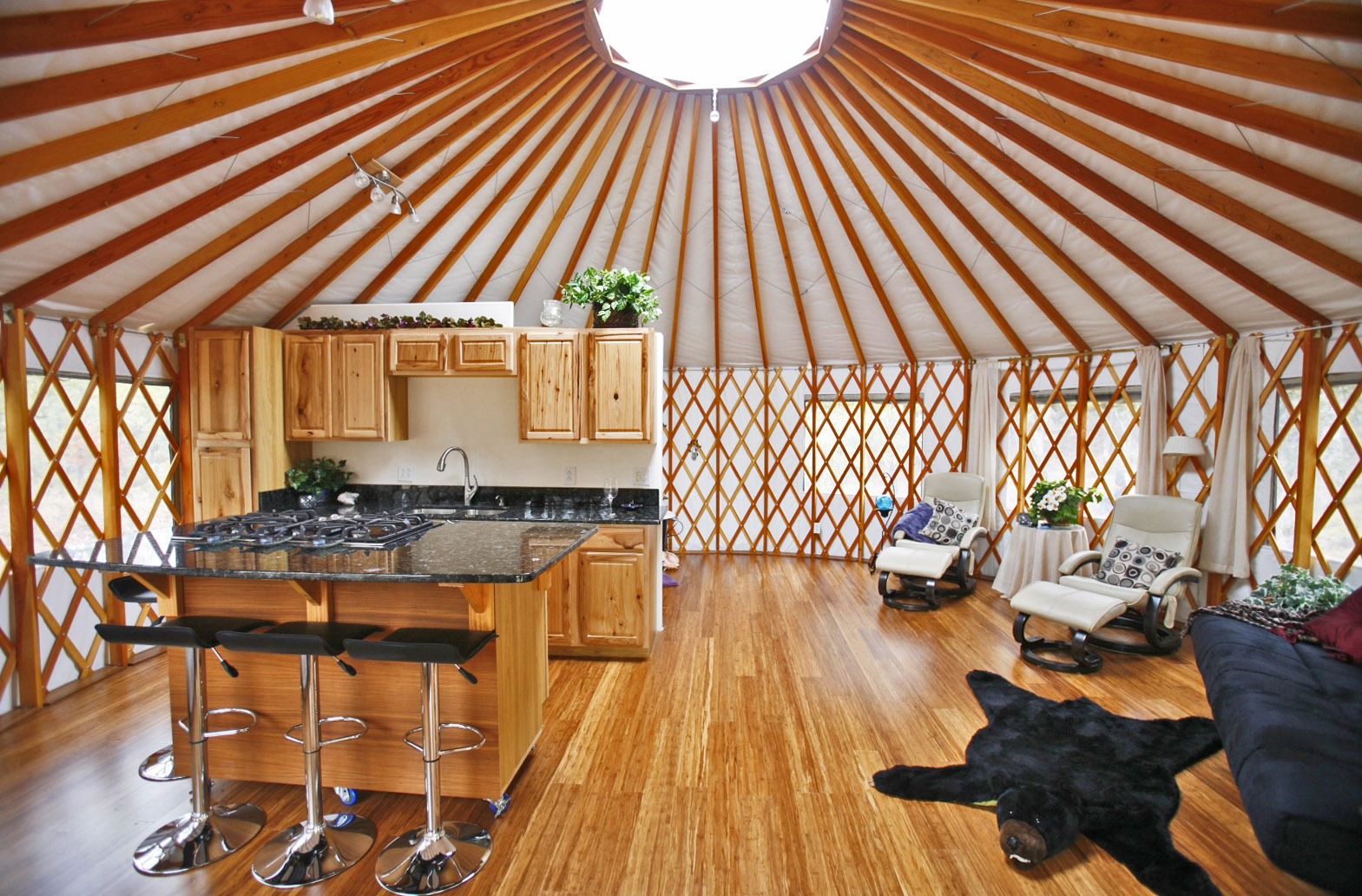The image portrays the interior of what appears to be a yurt, featuring a distinctive tent-shaped, circular roof that peaks at the center, adorned with a large central light. The spacious interior includes a combination of rustic and modern elements. Wooden flooring covers most of the area, punctuated by a striking skinned bearskin rug near the bottom right corner. On the left side of the image, a well-equipped kitchen area boasts wood cabinets, a sink, a faucet, an oven range, and an island with a black marble countertop, accompanied by three black and silver bar stools. Adding to the décor, a lattice-like section is visible over the windows. To the right, two white and black lawn chairs and a black futon provide a cozy seating area. This eclectic mix of features creates a unique and inviting atmosphere within the yurt.